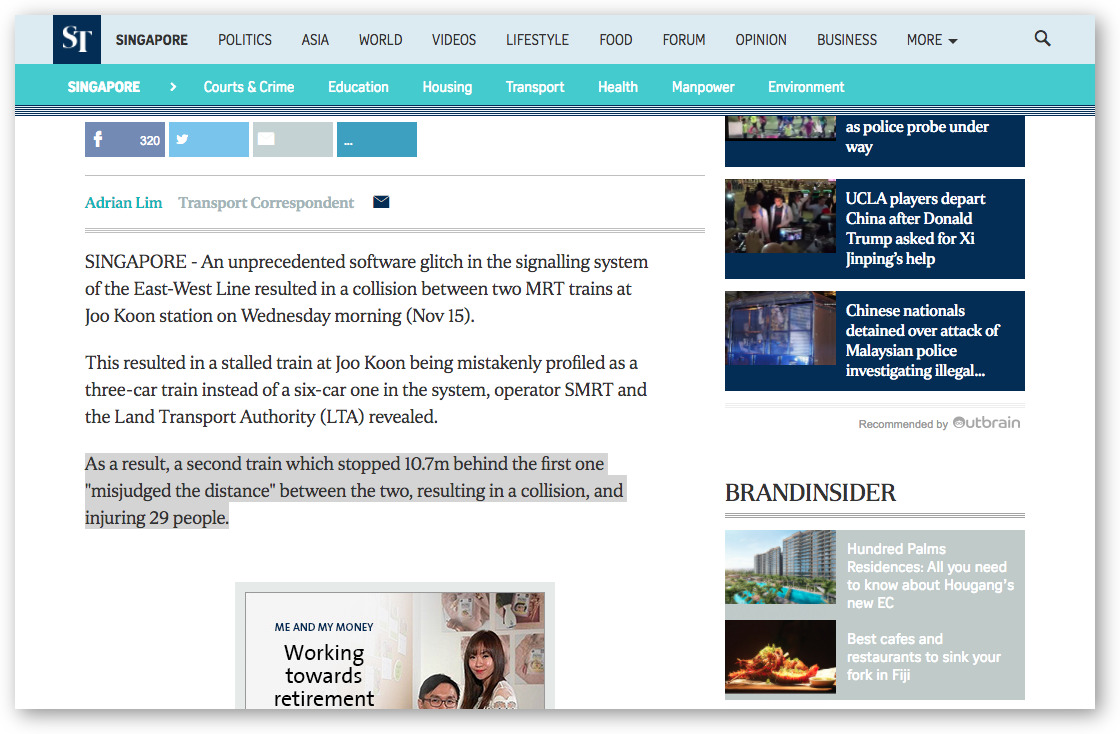The image depicts a detailed view of a Singaporean news website, which appears to focus on a broad range of topics. The top section of the website features a light blue banner with the site’s name, "Singapore," prominently displayed. Accompanying the site name is a comprehensive navigation menu offering categories such as Politics, Asia, World, Videos, Lifestyle, Food, Forum, Opinion, Business, and a drop-down menu with additional options.

Directly beneath this banner is another, colored teal, which again reiterates the name "Singapore" and includes another set of menu options specifically targeting Courts and Crime, Education, Housing, Transport, Health, Manpower, and Environment.

The main content visible in the image showcases an article pertaining to a significant incident involving Singapore's MRT system. The text begins mid-article, detailing a report about an unprecedented software glitch in the signaling system of the East-West Line. This glitch led to a collision between two MRT trains at the Joo Koon station on the morning of Wednesday, November 15. According to the article, the glitch caused a stalled train at Joo Koon to be incorrectly registered as a three-car train instead of a six-car one within the system. This misinformation led to a second train, which had stopped 10.7 meters behind the first, to misjudge the distance, resulting in a collision that injured between 26 to 29 people.

The article concludes with a highlighted paragraph - shaded in gray - that underscores the critical details of the incident. This paragraph summarizes the sequence of errors and the resultant injuries from the collision, emphasizing the severity of the incident.